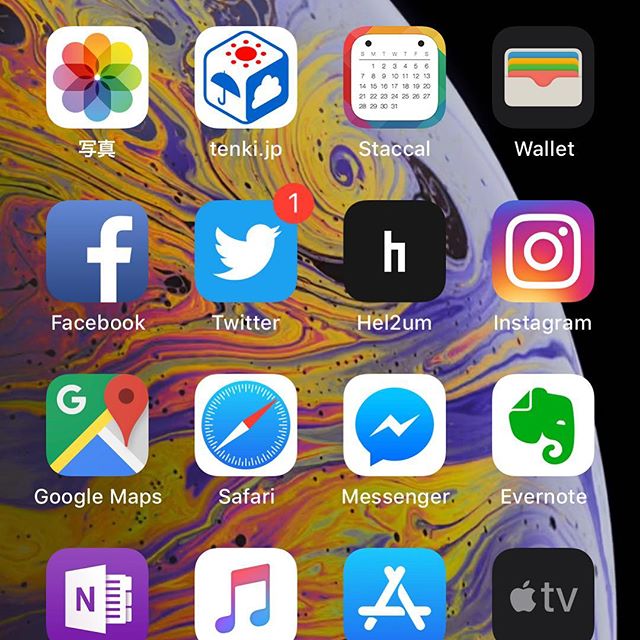This is a detailed description of a mobile phone screenshot featuring a vibrant, multi-colored marble wallpaper with purple, yellow, and orange swirls. The screen displays four rows, each containing four application icons, totaling 16 icons.

### First Row:
1. **Unknown App with Chinese Characters**: This app icon has a white background adorned with colorful flower petals, each a different color, surrounding Chinese characters.
2. **Unknown App with Dice**: The second icon has a design featuring dice with three faces—an umbrella, a cloud, and a sun symbol marked 'tanky GP'.
3. **Calendar App**: The third icon is a traditional calendar displaying an entire month with 31 days.
4. **Wallet App**: The fourth and final icon in this row is a wallet application.

### Second Row:
1. **Facebook**: The familiar blue and white Facebook icon.
2. **Twitter**: The blue bird icon that represents Twitter.
3. **Helium**: Next in line is the Helium icon.
4. **Instagram**: The colorful Instagram camera icon.

### Third Row:
1. **Google Maps**: Represented by the map and location pin icon.
2. **Safari**: The second icon features the compass of Apple's Safari browser.
3. **Messenger**: Facebook Messenger icon depicting a speech bubble with a lightning bolt.
4. **Evernote**: The green elephant logo of the Evernote note-taking app.

### Fourth Row:
1. **Unknown (Partially Visible)**: The first icon appears to be clipped in the screenshot and is mostly obscured.
2. **Unknown (Partially Visible)**: The second app icon is also only partially visible, making it hard to identify.
3. **Unknown (Partially Visible)**: The third icon follows the same pattern as the previous ones, being only partially visible.
4. **Unknown (Partially Visible)**: The fourth and last icon in this row is also partially visible, and its identity remains unknown.

This detailed description offers a thorough examination of each icon and provides insights into the wallpaper design and the visual layout of the mobile phone screen.